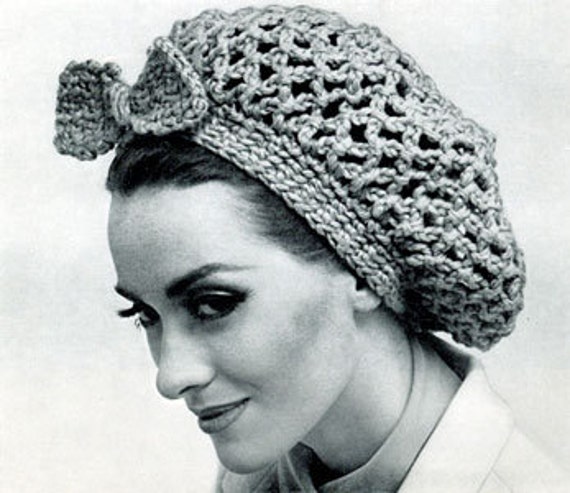This is a detailed black and white front-facing headshot of a striking model who bears a strong resemblance to Twiggy, the iconic English model from the 1960s. The image has a vintage style, yet it might be a modern recreation of a retro fashion. The model is adorned in a woollen crocheted beret-style hat with an intricate lattice pattern and an attached big crocheted bow at the front. Her dark hair is tucked neatly under the hat, emphasizing her expressive face. Her eyes are heavily made-up with prominent eyeliner and a smoky shadow, accentuating her large eyes. She has well-arched, neatly tweezed eyebrows, high cheekbones lightly highlighted with blush, and full lips wearing lipstick. Though her head is tilted down demurely, she looks shyly upwards at the camera with a charming smile. The model is dressed in a darker blouse that buttons at the collar, layered with a light-colored suit jacket. The overall composition and styling evoke the grace and elegance reminiscent of the 1960s fashion era.